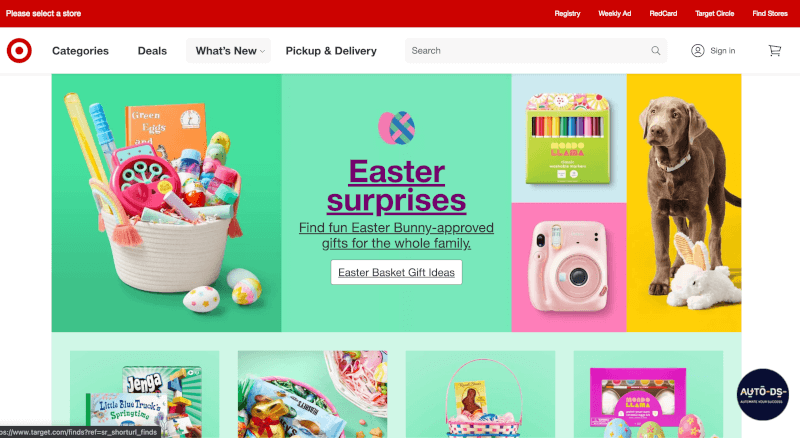The image depicts the homepage of an online store. The store's logo resembles an aiming circle, with a wide outer circle outlined in red and a smaller red circle at the center. A red bar sits at the top of the page, with the store's name, "Key Selector Store," written on the left.

On the right side of the red bar, various options are listed: "Regular Tea," "Weekly Ad," "Red Card Tiger Circle," "Feed Food Stores." Further down, navigation links are available for "Categories," "Deals," "What's New," "Pickup and Delivery," and a "Search" function.

The central part of the image features an Easter-themed basket filled with various goodies. Visible items include colorful Easter eggs positioned to the side, a pink toy clock, an orange book, a blue bubble blower with a transparent bottle, and a yellow elongated tool. The text accompanying this section reads: "Easter Surprises: Find Fun Easter Bunny Approved Gifts for the Whole Family, Easter Basket Gift Ideas."

To the right, there is another section displaying a small camera, crayons, a toy puppy wearing a name tag, and a stuffed rabbit doll. At the bottom of the image, additional pictures are partially visible, featuring what appear to be more Easter-themed items such as Easter eggs, chocolates, and bunny-shaped gold chocolates.